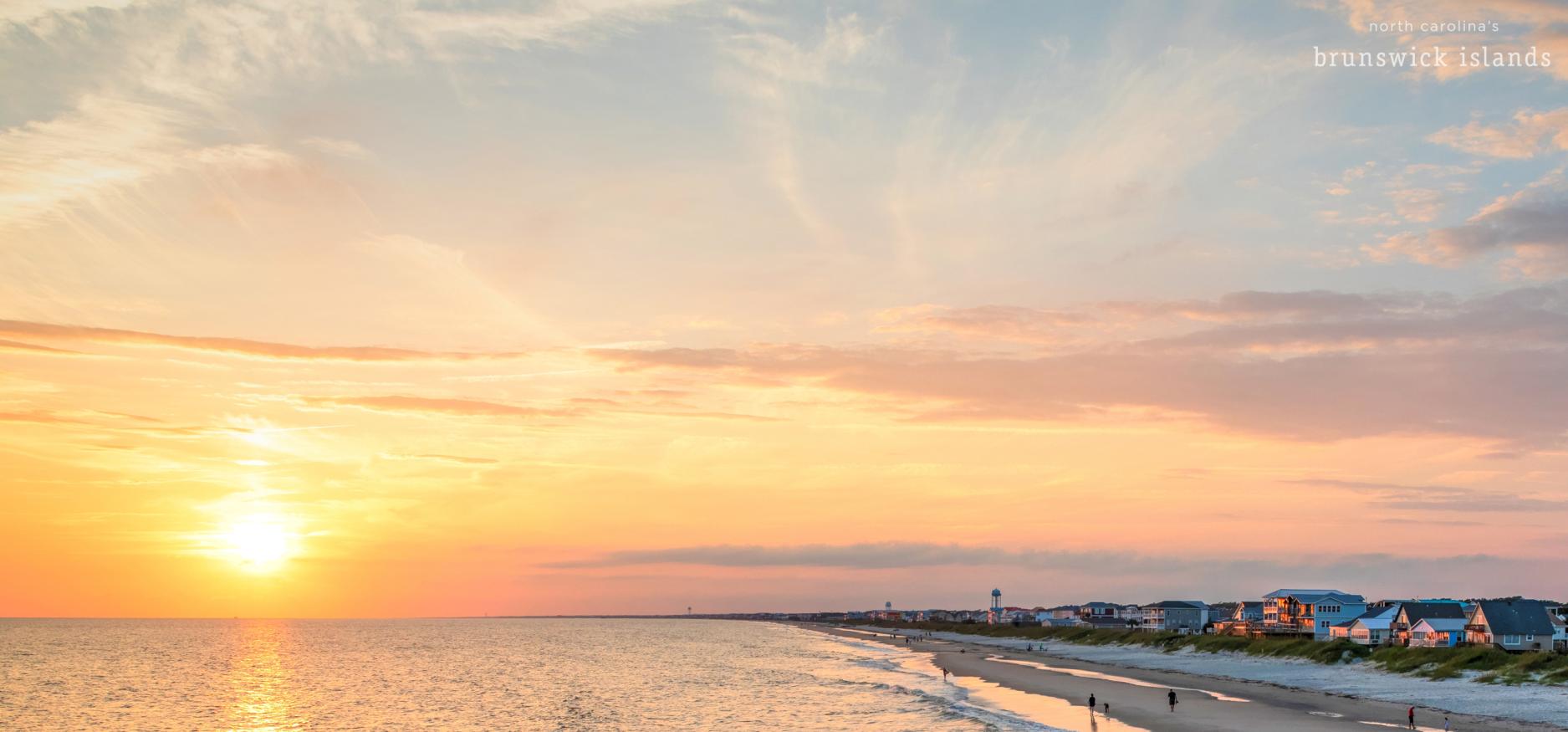This photograph captures a stunning sunset over the ocean, taken from a high elevation—likely from a drone—offering a high-angle view. The sky is a vibrant mix of diffused colors, transitioning from deep oranges and yellows near the horizon to purples and blues at higher altitudes, with a few scattered clouds. Below, the beach stretches out to the right side, dotted with sparse vegetation and lined with residential homes, some on stilts, extending to the very edge of the sand. A few people, small and ant-like due to the distance, stroll along the beach. A sign in the top left corner reads "North Carolina's Brunswick Islands,” confirming the location near the Outer Banks.